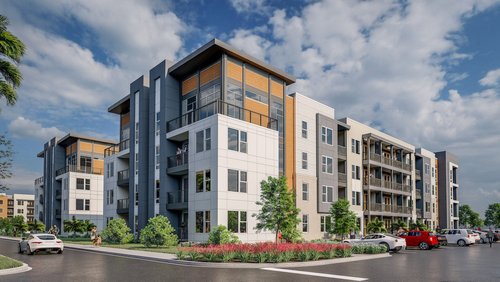Against a backdrop of a beautiful blue sky adorned with white, rolling clouds, a modern apartment or condo building stands prominently at a corner intersection. This freshly constructed building showcases a diverse color palette with white, tan, gray, and medium brown wooden panels accentuating the windows. The structure spans four floors and features several balconies that overlook a parking lot filled with cars, including a noticeable white sports car, a red car, another white car, and several other vehicles.

In the foreground, a flower bed bursting with pink flowers, possibly tulips, adds a touch of nature at the corner leading to the parking lot. Trees and bushes, including a distinctive palm tree on the left, surround the buildings, providing natural scenery and shade. The street, still glossy as if it had just rained, reflects the movement of a white sports car driving down the left-hand side. On the sidewalk in the bottom left corner, a woman and a little girl can be seen walking, adding a touch of life to the serene urban scene. The image captures not just one structure but a series of similar buildings extending into the background, creating a cohesive and vibrant residential area.